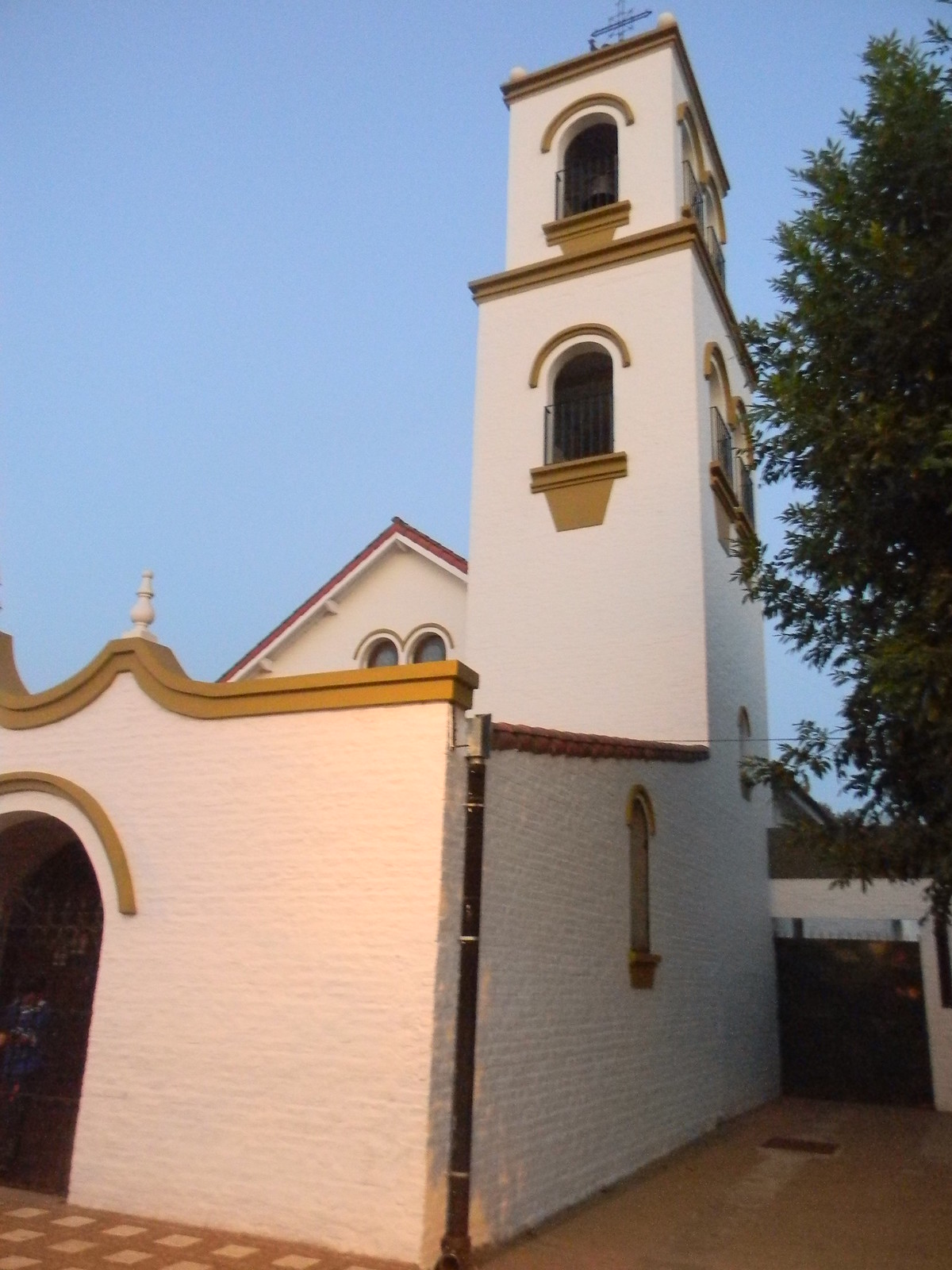This somewhat faded color photograph, likely taken close to dusk, captures an outdoor scene featuring what appears to be a white stucco church with brown accents, including wooden borders at the top and beneath the windows. The sky is notably clear but dimly lit, suggesting the light is fading. The ground is adorned with decorative, checkered tiles in shades of brown.

The church boasts a three-story tower, also white with gold decorative trims around several domed, arched windows, extending up the tower. A rounded doorway is visible in the lower left-hand corner, bordered by brown wood. A prominent metal gate is in the bottom left corner, while another fence extends from the right side of the building.

Also notable in the scene are a couple of green trees, with one large tree on the right side reaching the height of the third story. The overall impression is of a serene architectural landmark set against the backdrop of waning daylight.